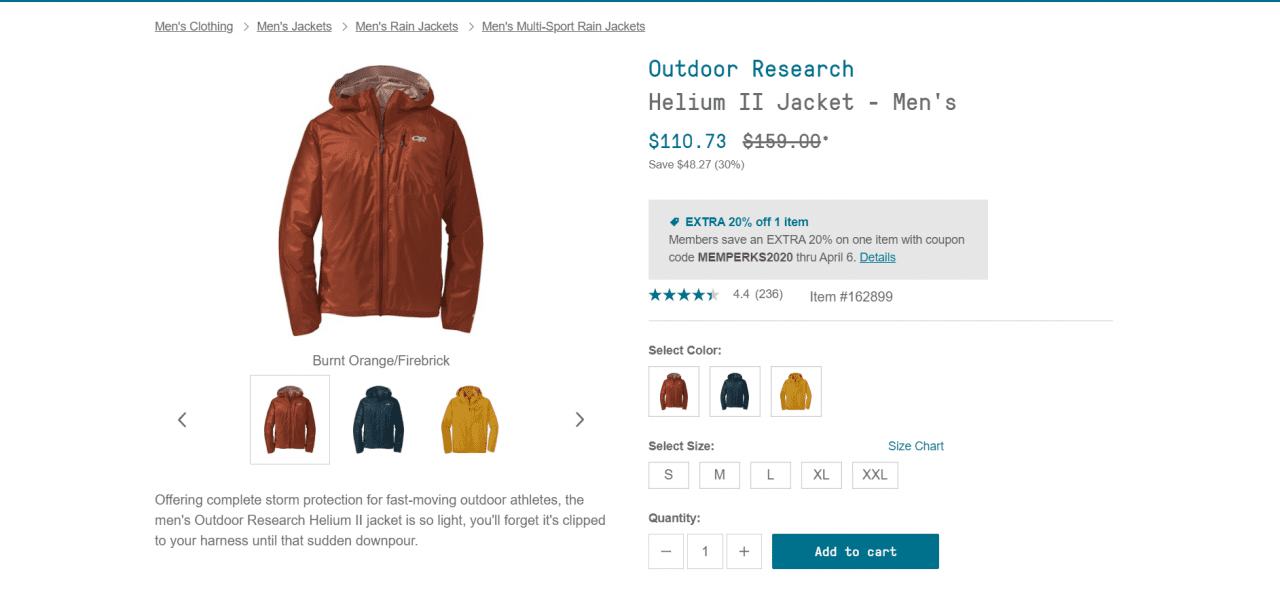This is an advertisement for the Men's Outdoor Research Helium 2 Jacket. The top left corner of the screen features navigation links: Men's Clothing, Men's Jackets, Men's Rain Jackets, and Men's Multi-Sport Rain Jackets. Dominating the center of the screen is an image of the Helium 2 jacket, showcased in a light to mid-brown color with a zip-up front and an attached hood. A small logo appears in white lettering on the right side of the jacket as viewed from the image. The text below identifies the color as "Burnt Orange/Firebrick."

Beneath the main image, there are three smaller thumbnails displaying the jacket in three different colors: burnt orange, blue, and yellow. Below these images, a small font caption states, "Offering complete storm protection for fast-moving outdoor athletes. The Men's Outdoor Research Helium 2 jacket is so light, you'll forget it's clipped to your harness until that sudden downpour."

On the right-hand side of the image, the text "Outdoor Research" is presented in blue, followed by "Helium 2 Jacket Men's" in grey. The price is prominently displayed in blue text as $210.73, with the original price of $150.00 shown in black text and crossed out.